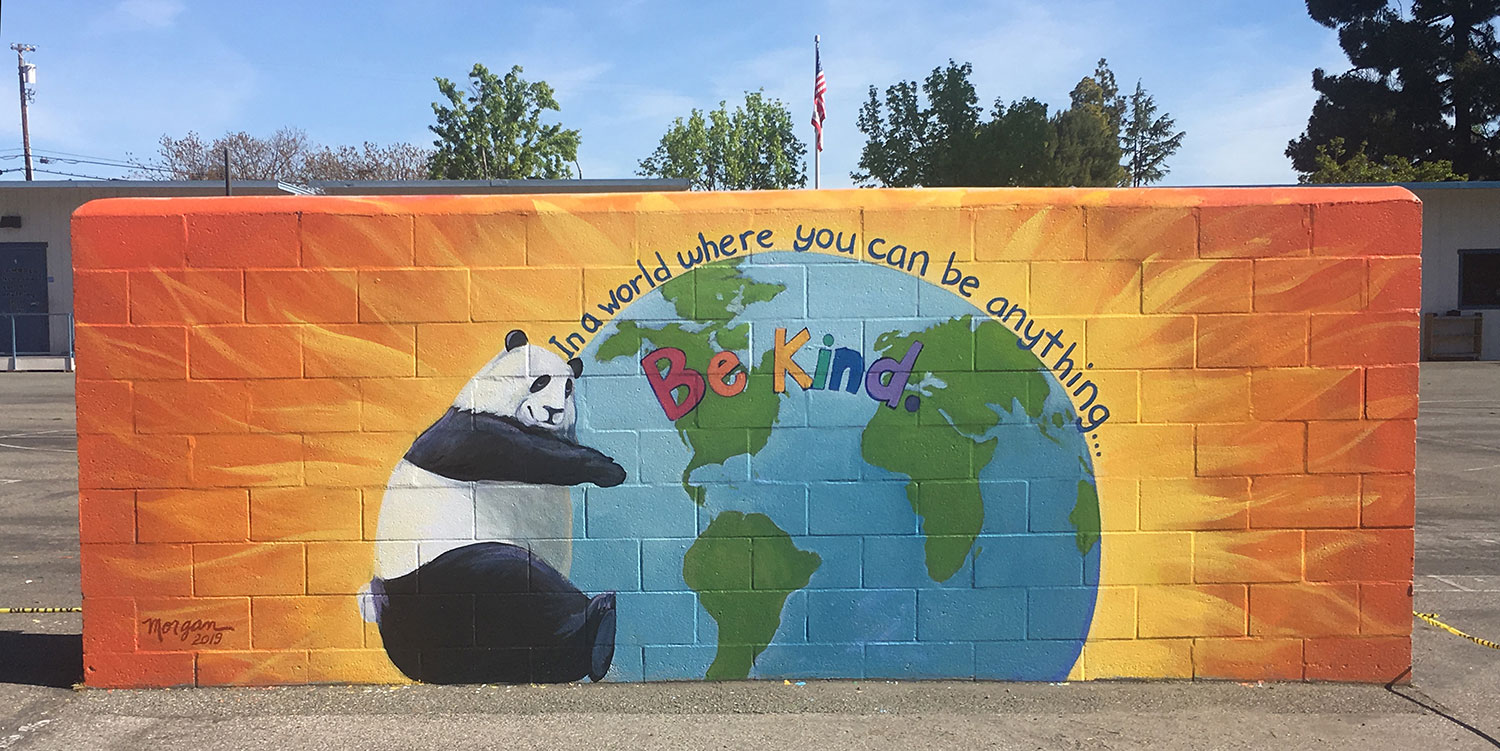This photograph showcases a vibrant piece of wall art painted on a concrete block wall in a parking lot. The wall, built of concrete blocks, is prominently painted in bright orange with sunburst gold accents around the edges. Central to the artwork is a vivid depiction of the Earth, with green continents and blue-green oceans. Inscribed over the Earth in multicolored lettering are the words "Be Kind," with each letter in pink, orange, green, blue, and purple. Above this, in blue letters, it reads, "In a world where you can be anything, be kind."

The Earth is affectionately embraced by a large panda bear on the left side, depicted with a white head, black arms, and a white midsection. The panda appears lovingly cradling the globe with its head resting against it and limbs wrapped around protectively. The mural is signed "Morgan, 2019."

In the background of the scene, a light blue sky with sparse white clouds stretches across the horizon, punctuated by an American flag visible in the distance. We also see a mixture of large and small trees and the partial view of a white building with a blue door amidst the greenery. Stripes marking the parking lot ground contribute to the setting, enhancing the contrast between the vivid mural and its surrounding environment.